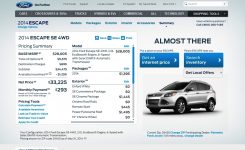This screenshot showcases a section of a car-buying application, specifically one provided by Ford. The interface appears to be part of a car configuration tool where users can customize their desired vehicle. Dominating the center of the screen is an illustrated car, although the specific model isn't discernible. On the left side of the screen, there is a densely packed column of small text likely detailing various configuration options and features available for customization. At the top of the interface, the text "Almost there" is clearly visible, suggesting that the user is close to finalizing their car configuration.